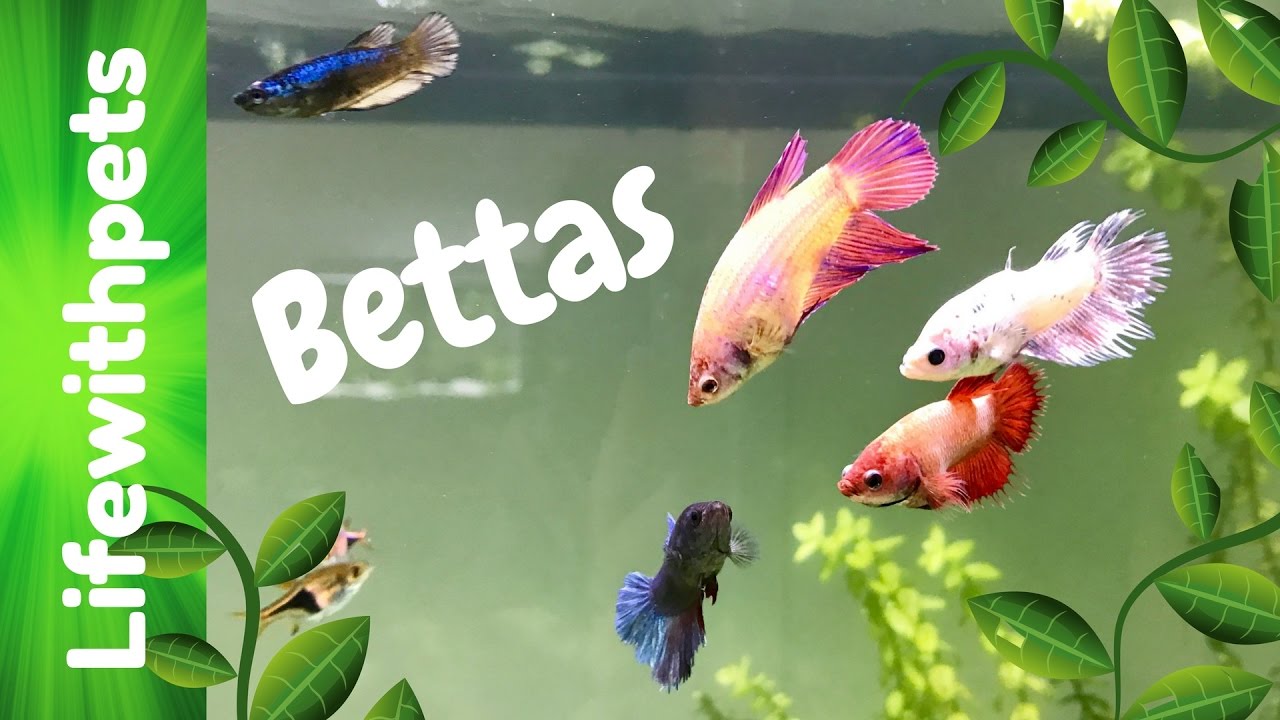The detailed graphic art depicts a vibrant fish tank teeming with vividly colored bettas and life-like details. The background water is a calming blue, and alongside the tank glass, the words "Life with Pets" and "Bettas" stand out in bold, white lettering.

The tank is lushly adorned with various green leaves, some of which are sprinkled with lighter green veins. These leaves occupy the left side, extend up the right side, and partially cover the bottom right corner. There are also a few real yellow-tinted leaves interspersed, adding an extra layer of authenticity.

Center stage in this aquatic scene are several striking betta fish. A blue fish with a silver hue and black markings swims near the top left, while in the middle, a prominent pink fish with matching fins and tail captures attention. Below this pink betta is a white fish with equally pristine fins and tail. Descending further, a predominantly red fish with a pink body boasts vivid red fins and tail. Close by is a purple betta, adding to the spectrum of colors. Other fish include those with combinations of black, clear, and bluish hues, each contributing to the lively display.

Completing this underwater tableau, white flowers and additional green leaves enhance the naturalistic feel, with some blossoms and stems seen throughout the tank. The meticulous arrangement and diverse colors create an engaging and life-like depiction of aquatic life.